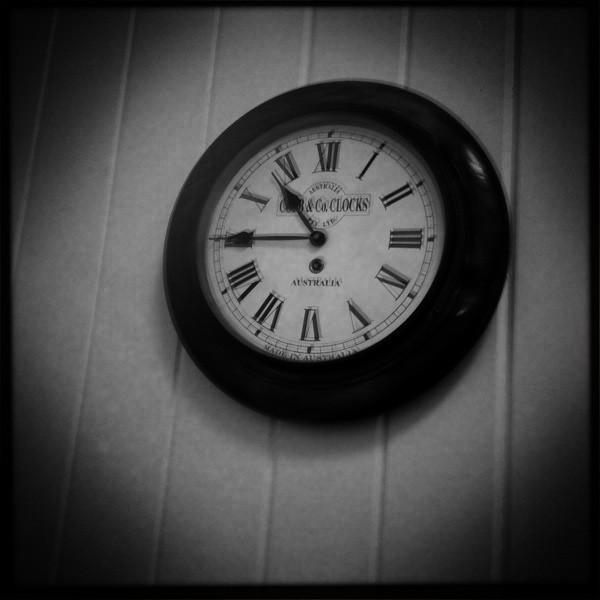The black-and-white image features a clock mounted on a wall, which appears to be made of vertically aligned wood paneling, possibly white or gray in color. The clock, positioned at the center of the photograph, is round with a prominent all-black border. The face of the clock, encircled by this border, is white and adorned with Roman numerals in black. Black hands indicate the time as 10:45. The inscriptions on the clock include "Cobb and Co Clocks" and "Australia" located just above the number six. The photo has a vignette effect, causing the corners to appear almost black, giving the impression of viewing through a peephole.